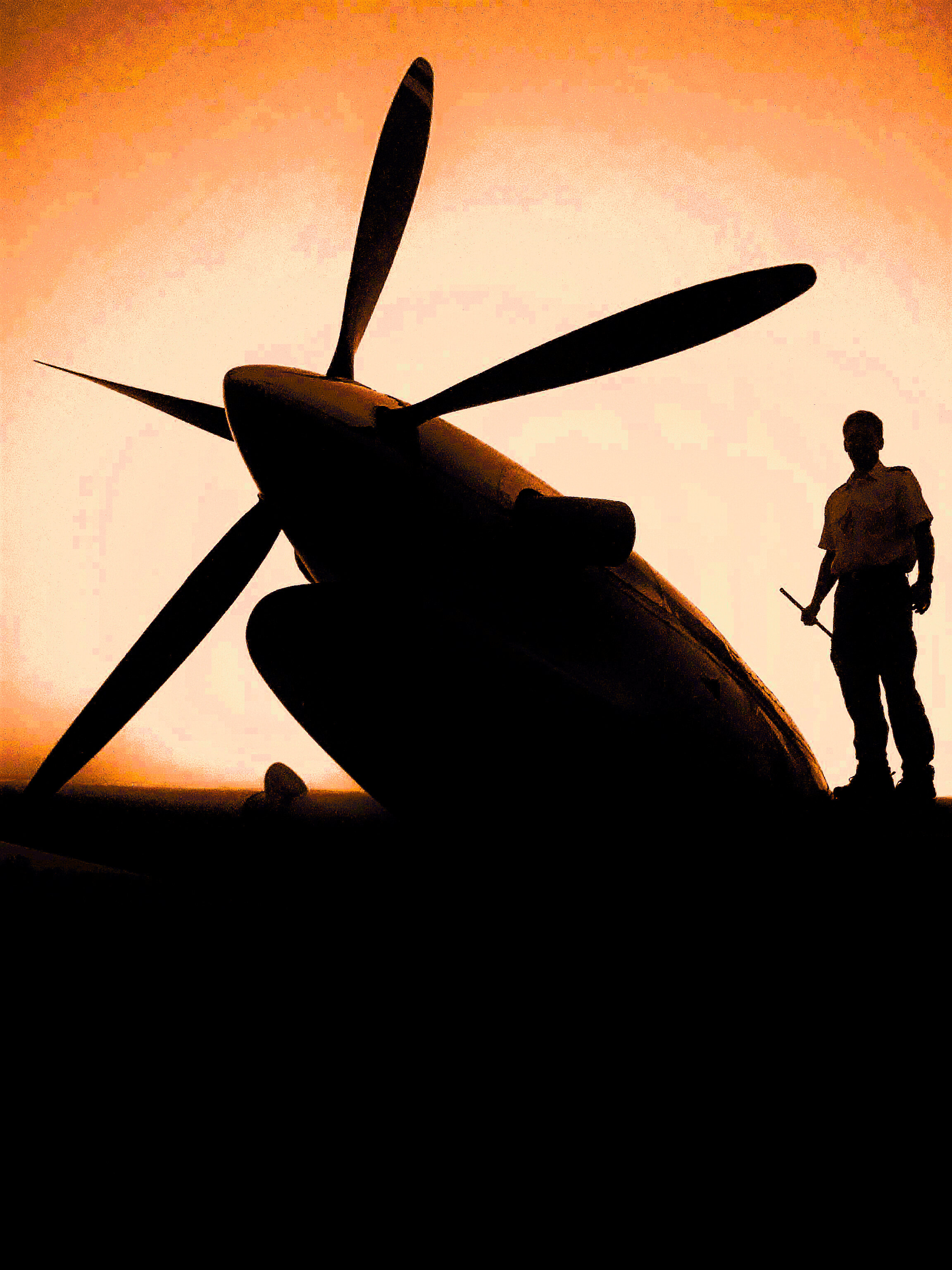In this striking image set against a vivid sunset, a man stands silhouetted on the wing of a World War II fighter plane. The sky transitions beautifully from a bright yellow at the horizon to deep orange tones as it ascends, creating a dramatic backdrop. The aircraft’s four-bladed propeller, which appears to have a shiny metal tip, is prominently featured, with the sun positioned directly behind it, enhancing its dark, pointed silhouette. The man, indistinguishable in details but clearly outlined in shadow, is dressed in a short-sleeved shirt, overalls with one strap, and boots. He holds a tool, possibly a wrench, in his right hand. The scene exudes a nostalgic atmosphere, capturing a moment that blends historical aviation with the quiet intensity of dusk.